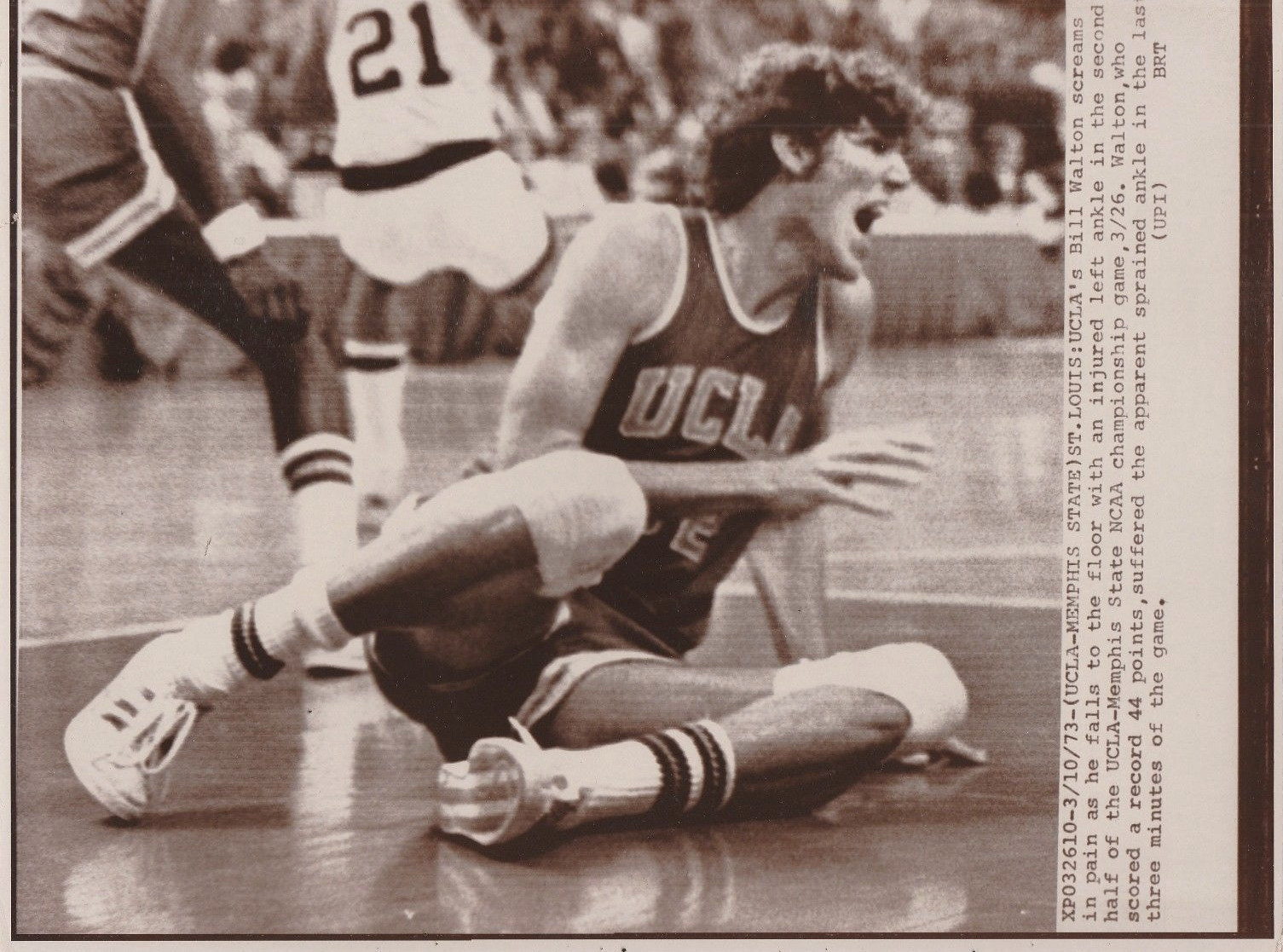This black-and-white image, resembling an old newspaper photo, captures UCLA basketball player Bill Walton on the ground, evidently screaming in pain from an injured left ankle during the UCLA vs. Memphis State NCAA championship game on March 10, 1973, in St. Louis. Walton, sporting a dark-colored UCLA uniform, has his face contorted in agony, providing no uncertainty about his distress. In stark contrast, a player from the opposing team, wearing a light-colored uniform with the number 21, is visible in the background. The accompanying text beside the image reads: "XP 0 3 2 6 1 0 - 3/10/73 - (UCLA - Memphis State) St. Louis - UCLA's Bill Walton screams in pain as he falls to the floor with an injured left ankle in the second half of the UCLA Memphis State NCAA championship game 326. Walton, who scored a record 44 points, suffered the apparent sprained ankle in the last three minutes of the game. (UPI, BRT)."